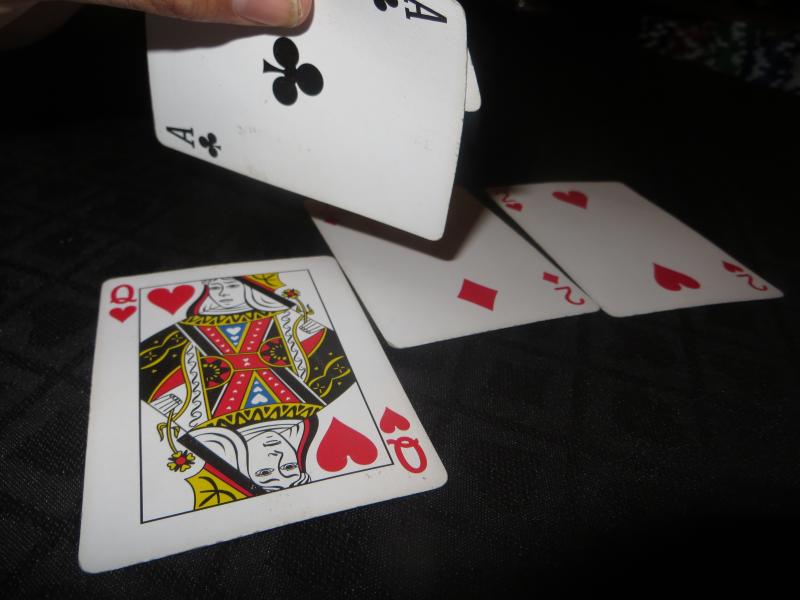The color photograph captures a moment in a card game, illuminated by a flash or an overhead light source positioned over the left shoulder of the viewer. The background is a stark black, highlighting the scene on what appears to be a glass tabletop. Below the surface, a checkerboard or windowpane patterned rug is partially visible.

In the image, a thumb entering from the top left is holding an Ace of Clubs and another not visible card, seemingly about to lay them down on the table. On the table already are three face-up cards: the Queen of Hearts, the Two of Diamonds, and the Two of Hearts. The two twos are positioned side by side, while the Queen of Hearts occupies most of the lower left-hand side of the photo, closest to the camera. 

Due to the perspective, the Queen of Hearts appears slightly distorted, with one end looking larger and the other narrower. In contrast, the two twos lie flat, maintaining their proper proportions. The photograph captures the intensity and anticipation of the card game in progress.